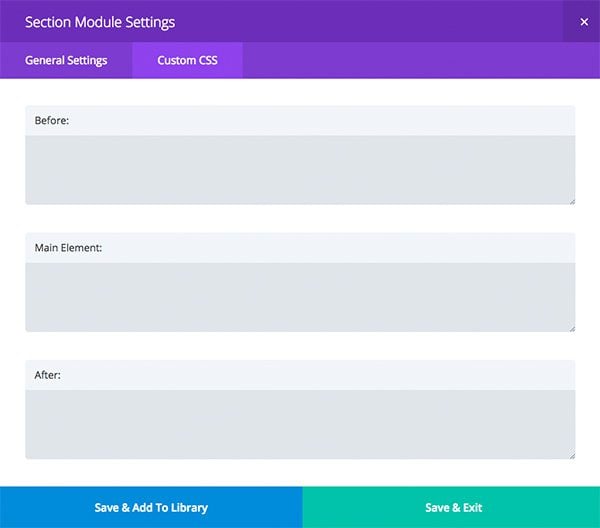Screenshot of a "Section Module Settings" Interface:

- **Top Section**: 
    * A prominent purple bar at the top displaying "Section Module Settings" in bold, white text.
    * To the right, a white "X" icon allows you to close the screen.

- **Second Section**: 
    * Below the top bar is a lighter purple bar labeled "General Settings" in white text.
    * Highlighted adjacent to it is a tab labeled "Custom CSS".

- **Content Area**: 
    * There are three expandable input sections:
      1. **Before**:
          - A text input area for custom CSS code that can be expanded by clicking the lines in the lower right corner.
      2. **Main Element**:
          - Similar to the first, a text input area for custom CSS that features expandable lines in the same location.
      3. **After**:
          - Another expandable text input area following the same format as the above sections.

- **Bottom Section**:
    * Two buttons for saving:
        - A medium blue button labeled "Save & Add to Library".
        - An aqua blue button labeled "Save & Exit".